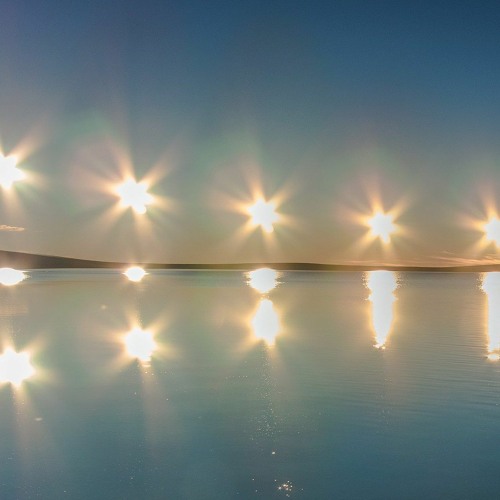The image captures a tranquil scene where a blue-green body of water meets the horizon under a sky that straddles the line between night and dusk. Five intensely bright lights, each arranged in a perfectly straight line and distanced equally from one another, pierce through the sky. These lights cast star-like glares with multiple points, their origins obscured by their own brilliance. The reflections of these lights dance upon the water below, some mirroring precisely while others stretch into elongated, distorted forms. A narrow, dark strip of land marks the horizon, void of buildings, and serves as a boundary between the still water and the expansive, deep blue sky. Little white spots pepper the lower parts of the water, adding texture to the serene expanse.